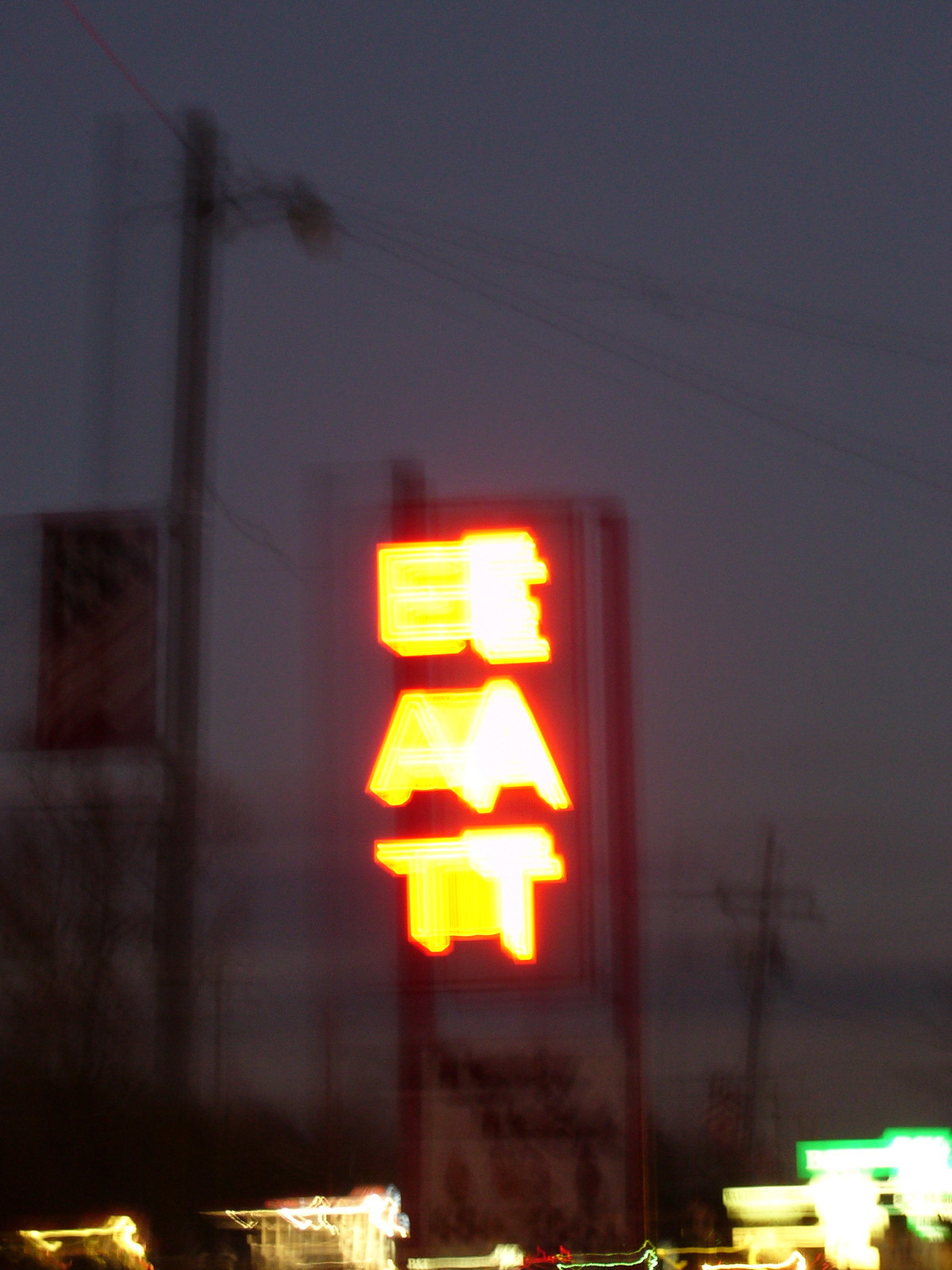The image depicts a nighttime urban scene engulfed in darkness, with a distinctly blurred backdrop. Dominating the background are two indistinct street poles, adding to the ambience of the city night. The focal point is a large advertisement signboard that stretches vertically, albeit shrouded in blur. The sign is divided into two columns of text; one features prominently bright yellow letters spelling out "E-A-T" from top to bottom, while the adjacent column repeats the same letters in white. Below this, the lower portion of the image captures a chaotic blur of street lights, buildings, and streets, suggesting either a high-speed photo capture or motion during the shot. The overall effect is a hazy, dreamlike snapshot of urban nightlife.